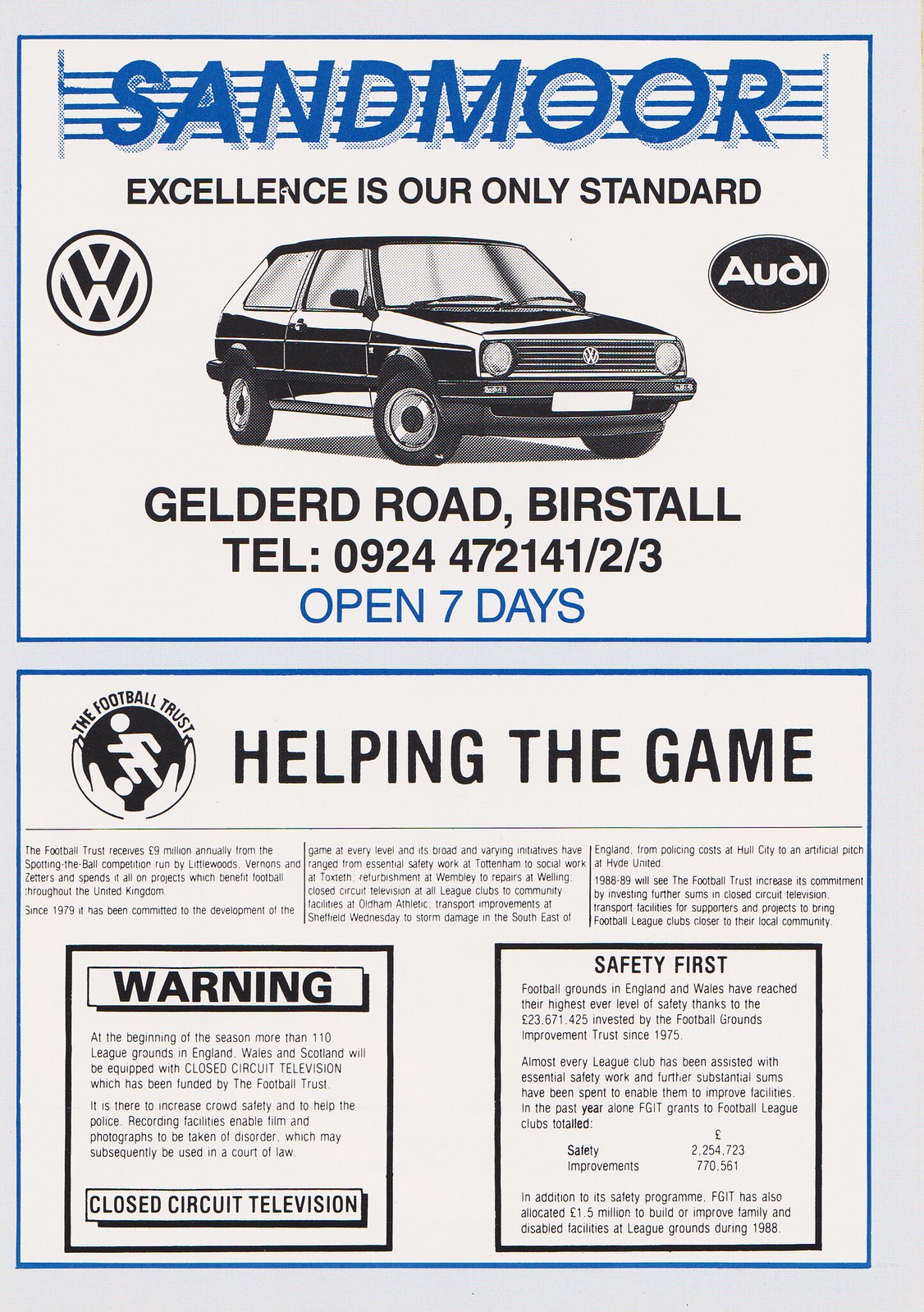The image is a detailed advertisement for a car dealership. It features a purplish, light blue background with a light gray border. At the top of the ad, in bold blue capital letters, it states "SANDMORE". Directly beneath, in black font, it reads "Excellence is our only standard." Below this text, there is a central image of a black and white station wagon flanked by the Volkswagen emblem on the left and the Audi emblem on the right.

Further down, in black text, the address "Gelderd Road, Bristol" is displayed along with the phone number "0924-472-141-2-3". In blue text, it notes that the dealership is "Open 7 Days". 

Beneath this, there is a smaller box containing additional information. On the left side, it says "The Football Trust" with a stylized image depicting hands holding a ball and a person running and kicking a ball. Accompanying text in blue reads "Helping the game". 

At the bottom, there is a warning sign about closed-circuit TV with some unreadable text and a safety notice that says "Safety First".